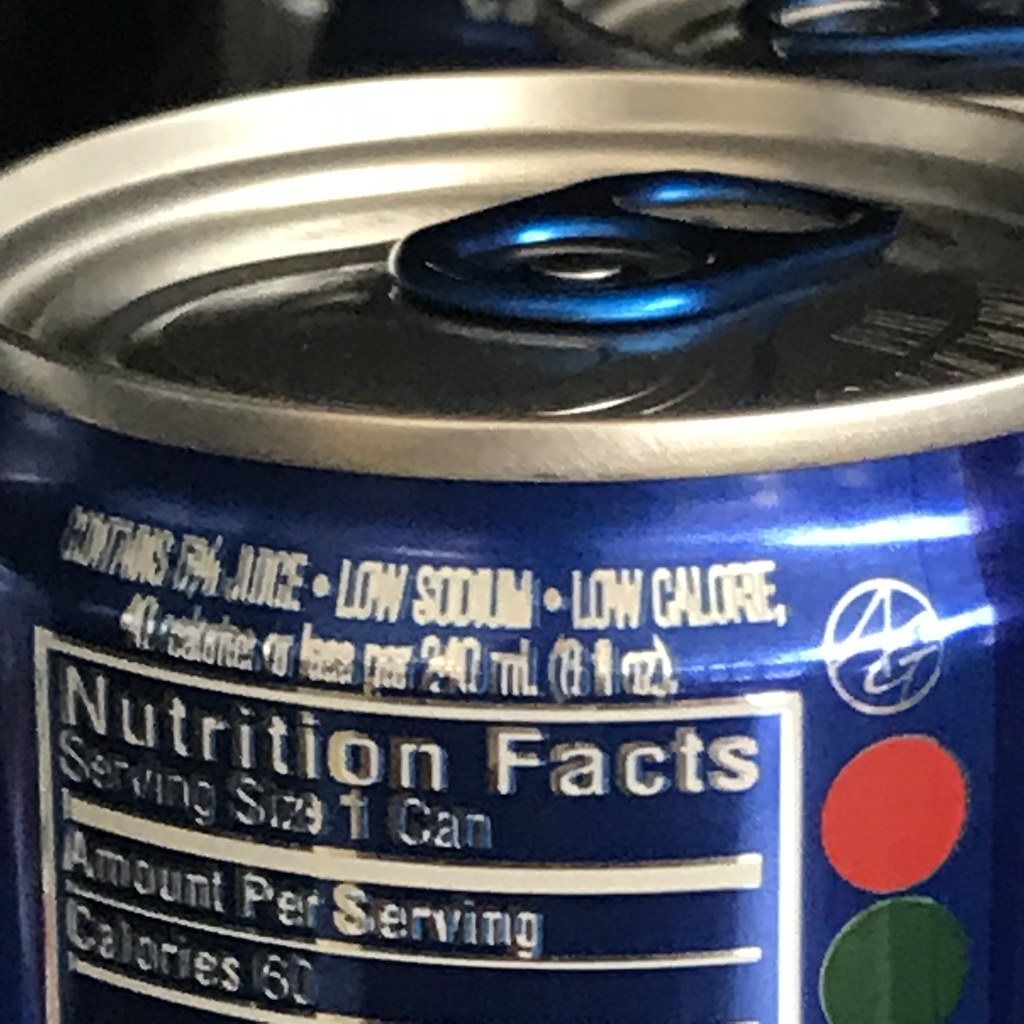This photograph depicts a sleek aluminum soda can with a metallic blue exterior. The top of the can is sealed, featuring a silver lid with a distinctive blue metallic pull tab. The front of the can prominently displays its key nutritional highlights in white text: it contains 5% juice, is low in sodium and calories, and provides 40 calories or less per 240 milliliters (8 fluid ounces). The nutritional information indicates a serving size of one can, with a total of 60 calories per serving. To the right, a logo consisting of the letters "AG" is visible, accompanied by a red dot above a green dot. The overall aesthetic of the can is modern and appealing, with a focus on health-conscious details.